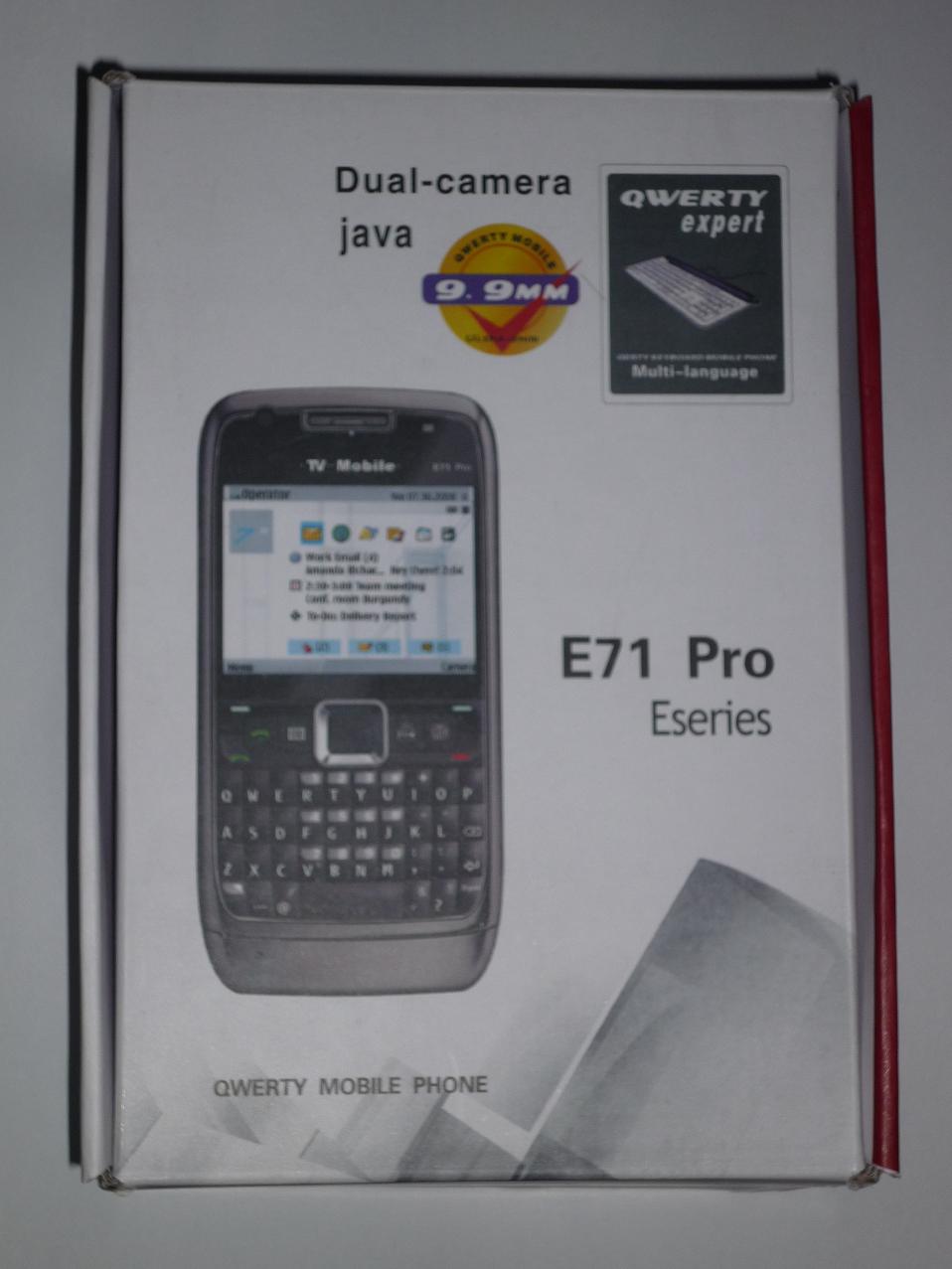The image depicts a product box for an older mobile phone labeled as "QWERTY Mobile Phone E71 Pro E-Series." The box prominently features an image of a phone with a small screen and a full keyboard below it, suggesting it is a QWERTY handset. A yellow circle logo with a red check mark is centered at the top, while a blue banner across the middle announces "9.9 mm." In the top right corner, there's a gray section with an icon of a keyboard labeled "QWERTY Expert Multi-Language," hinting at multilingual support. The box also mentions key features such as "Dual Camera," "Java," and "QWERTY Expert." With a predominantly white background and black text, the box's design reflects a style likely from the early 2000s, possibly around 2007. The brand name is unclear, but the emphasis on QWERTY and the model details are evident.